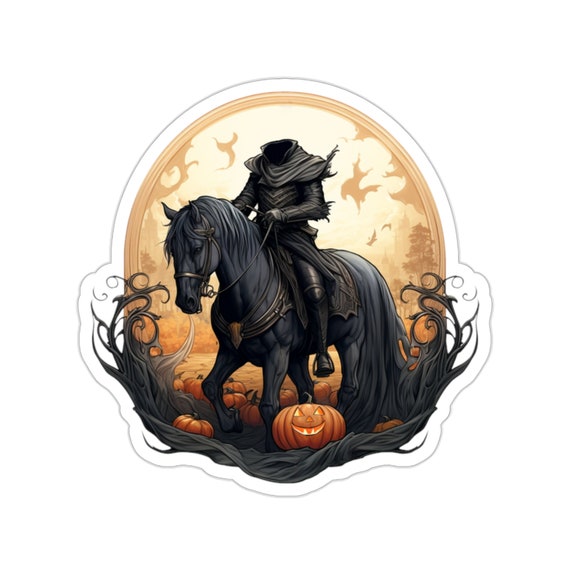This highly stylized, computer-generated drawing of the Headless Horseman has the feel of a high-quality sticker. Framed in a distinctive orangey-brown oval with intricate flourishes and dark brown, curling branches that extend halfway up each side, the image exudes a spooky, gothic atmosphere. At its center is an all-black headless horseman riding a matching black horse, turned slightly to the viewer's left. The horseman, depicted with slim, knight-like attire, complete with a long jacket, tights, and a scarf-like garment over his shoulders, grips the reins atop a saddle. The background subtly features vague images of birds and nature in a monochromatic scheme. Enhancing the eerie scene are scattered pumpkins along the bottom, including a jack-o'-lantern that stares out with a mysterious smile. Twisted tree parts frame the lower portion of the drawing, adding a final touch to its haunting aesthetic.